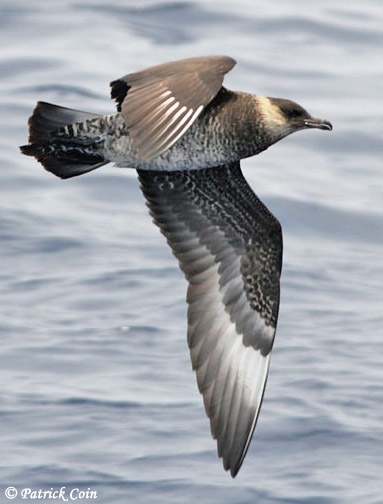In this captivating image, a Pomeranian Jaeger is captured mid-flight over a serene body of grayish-blue water, perhaps an ocean or sea. The bird, facing right, displays a dramatic wing posture: its left wing is extended low, almost touching the slightly rippled water, while its right wing is elevated close to its body. The bird's plumage features a striking combination of gray shades with a lighter underbelly and pronounced black and white modeling. Its head and beak are distinctly black, accented by a light stripe across its neck. The setting suggests a daytime photo shoot, with the natural hues of blue, gray, brown, and black blending harmoniously. In the bottom left corner of the image, the white text credits, "copyrights, Patrick Coyne," affirming his ownership and authorship of this stunning photograph.